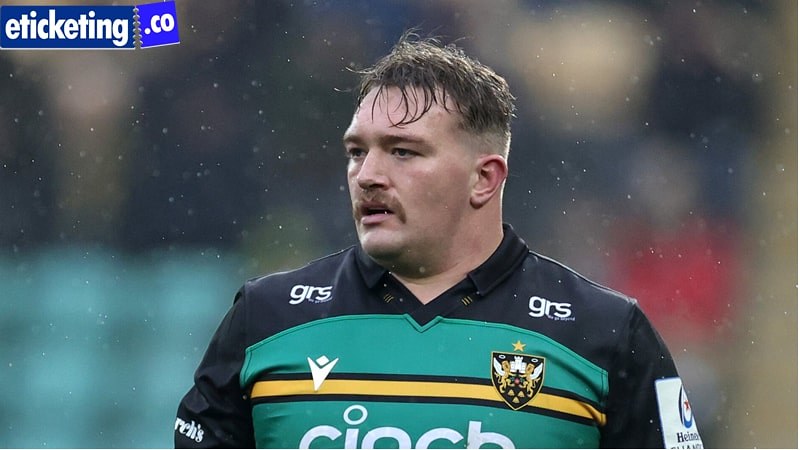This photo captures a male athlete as the main focus, with the background artistically blurred. In the upper left corner, there’s a box containing the text "eTicketing.co." The athlete, heavy-built with short hair that appears wet and stringy, possibly from sweat, also sports a mustache. He is dressed in a distinctive uniform, visible from the chest up. The uniform features black sleeves and shoulders, while the chest area is green adorned with a yellow stripe bordered in black. Prominently displayed on his chest is a shield logo depicting two lions holding a castle, along with a smaller human form logo with raised arms, and the white letters "GRS" near the shoulders. The overall scene suggests it might be snowing, adding to the dynamic atmosphere of the image.